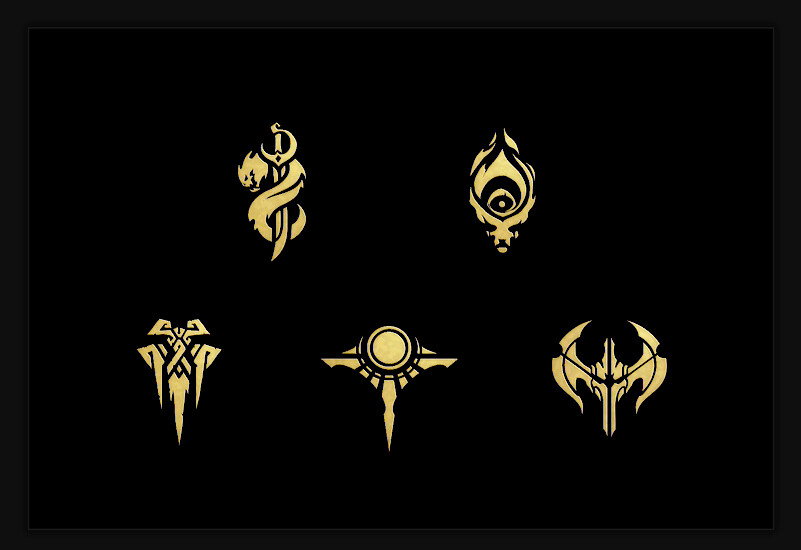On a pure black background, bordered by a lighter black frame, this image features five distinct gold emblems, organized in two rows with two on the top and three on the bottom. 

- The top left emblem is a sword pointing downwards, intricately wrapped with a serpent or dragon.
- The top right emblem depicts an eye engulfed in flames, evoking an evil eye on fire.
- On the bottom left, there's a circular design resembling a person flexing both arms, with a collar-like feature around the neck.
- The middle bottom emblem features a circular orb with beams extending from it, flanked by two silhouettes of dogs facing opposite directions, resembling a scepter.
- The bottom right emblem portrays a monstrous skull with cleaver-like blades jutting out from either side, resembling a warrior helmet with antlers.

Each emblem is rendered in gold, standing out starkly against the dark background.